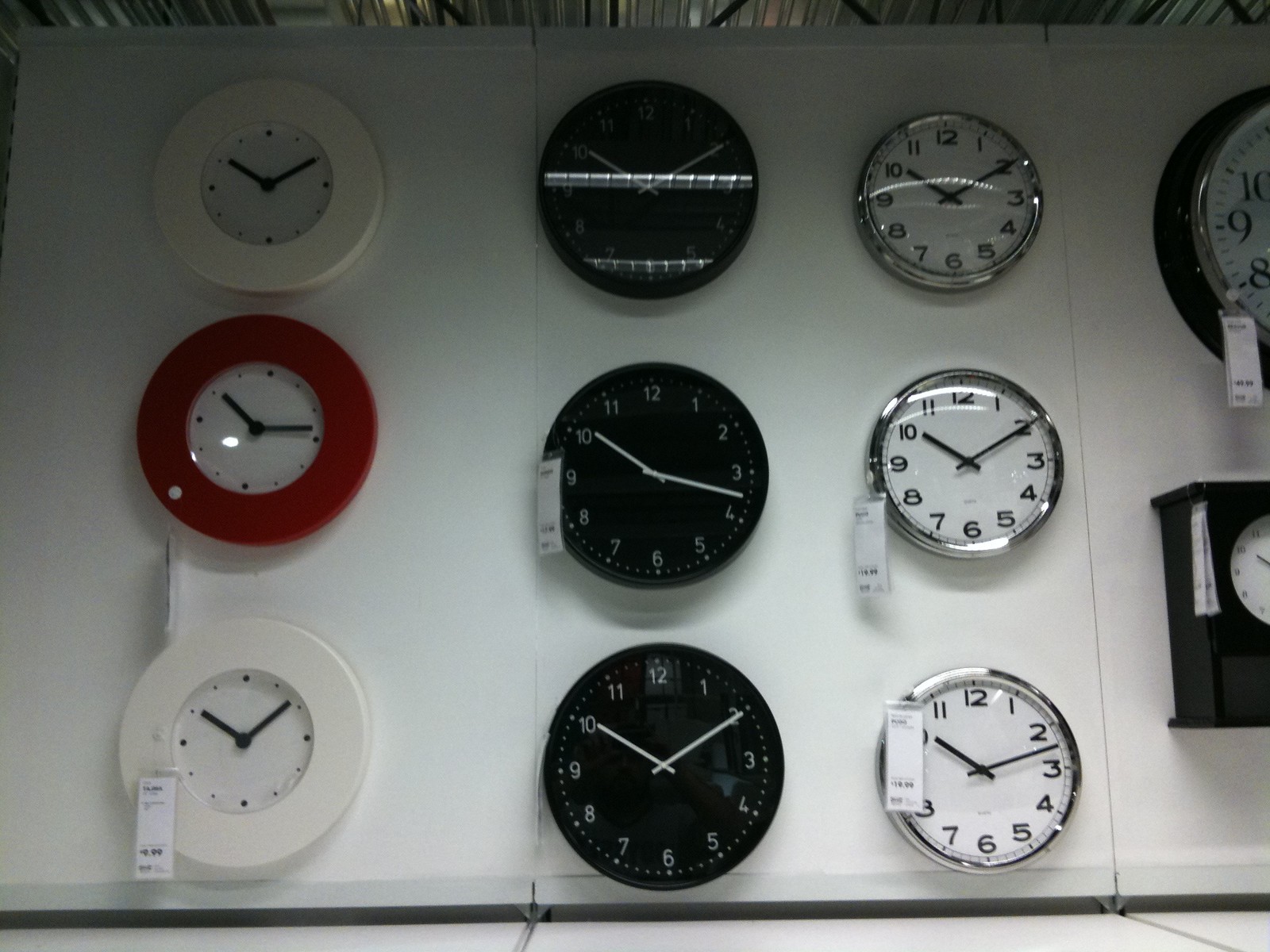This photograph captures a striking display of clocks arranged in a grid-like pattern on a white wall, with the visible portions forming three rows and three columns. There are nine fully visible, circular clocks, each showcasing a unique design and varying in color—some black, some white. Dominating the right side is a partially visible rectangular clock, standing out due to its distinct shape.

All the clocks display a time close to 10:10, but with slight variations. The clock on the bottom right reads around 10:12 or 10:13, the one in the center shows 10:17, and the clock on the left center indicates 10:14. Meanwhile, the clock on the top left appears to be slightly earlier than 10:10. These minor differences in time create an intriguing visual and temporal dynamic. The clocks' faces catch reflections, adding a layer of complexity to the image.